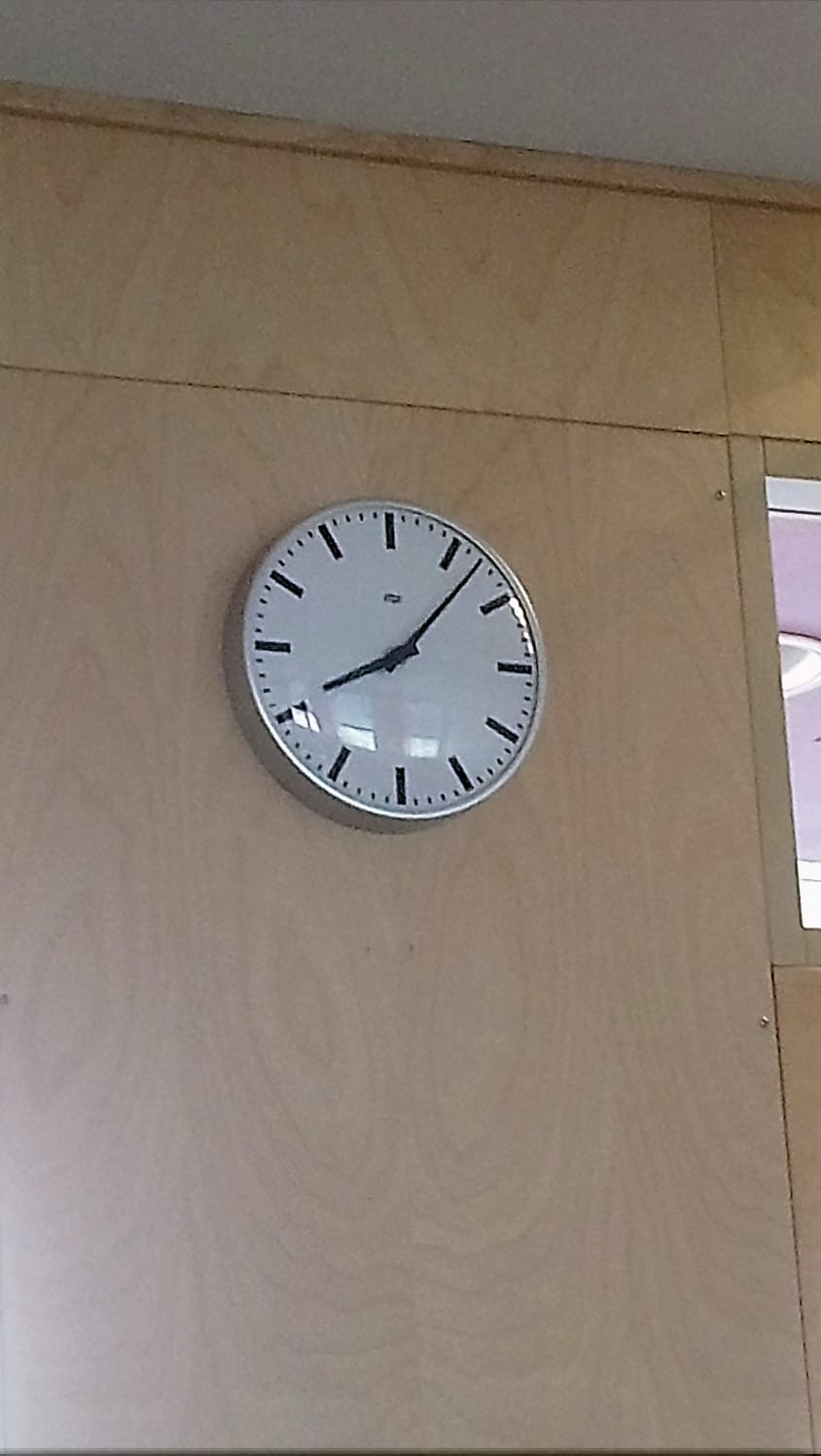This detailed photograph, oriented in portrait mode, captures the focal point of a modern, round wall clock positioned on a light-colored wooden wall that resembles a temporary partition panel. The clock is distinguished by its minimalist design, featuring a white face with black hands— a thin black minute hand and a slightly shorter, thicker hour hand—set against an absence of numbers. Instead, the clock face is marked by black dashes at each hour position, with smaller dashes denoting the minutes. Encased in a notably reflective, silver-colored rim, the clock's glass or plastic cover accurately reflects a series of windows behind the camera, indicating the photo was taken indoors during daylight hours. The time displayed on the clock is approximately 8:07. The top edge of the photograph includes a faint glimpse of the grey ceiling, and to the right, there's an ambiguous opening or window that allows light to filter through. This image is devoid of any human or animal presence, textual elements, or natural flora, maintaining focus entirely on the minimalist clock and its surroundings.